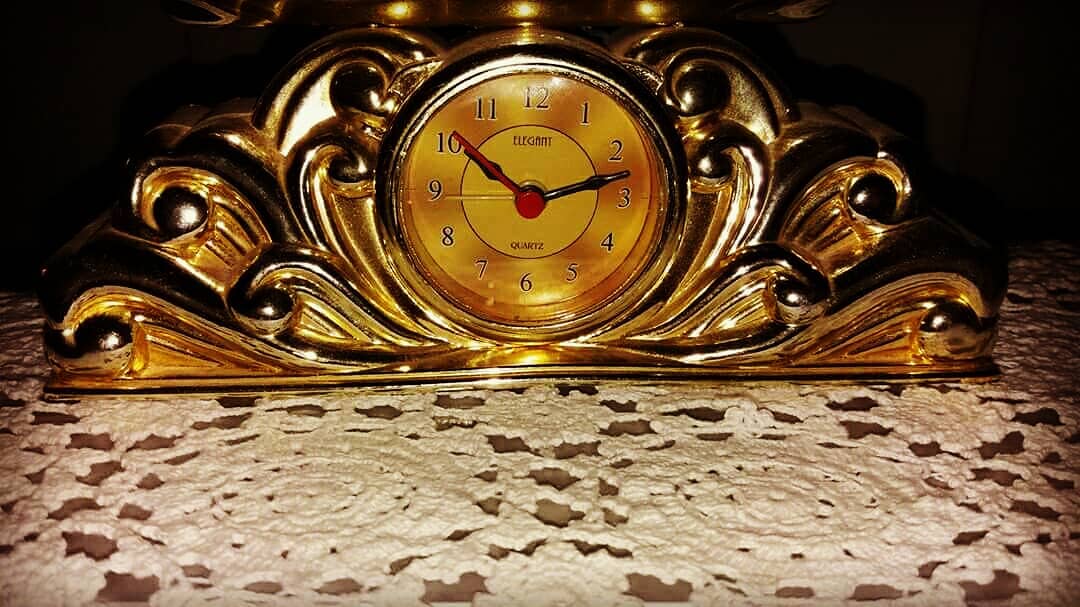This color photograph showcases a stunning, ornate tabletop clock with intricate details. The analog clock features a captivating gold face adorned with traditional numbers. It displays the time as approximately 10 minutes to 2, with distinct black minute and hour hands, complemented by a red sweeping second hand.

The clock is encased within an exquisite metal casing, which artistically extends on either side resembling petals. This design gives the impression of the clock being a flower with six petal-like extensions on both the right and left sides, crafted from a gold or gold-tone metal.

The clock is elegantly placed on a table adorned with a beautifully hand-crocheted, white lacy tablecloth, adding a delicate and refined touch to the overall composition. The craftsmanship of the tablecloth further enhances the elegance and charm of the scene.